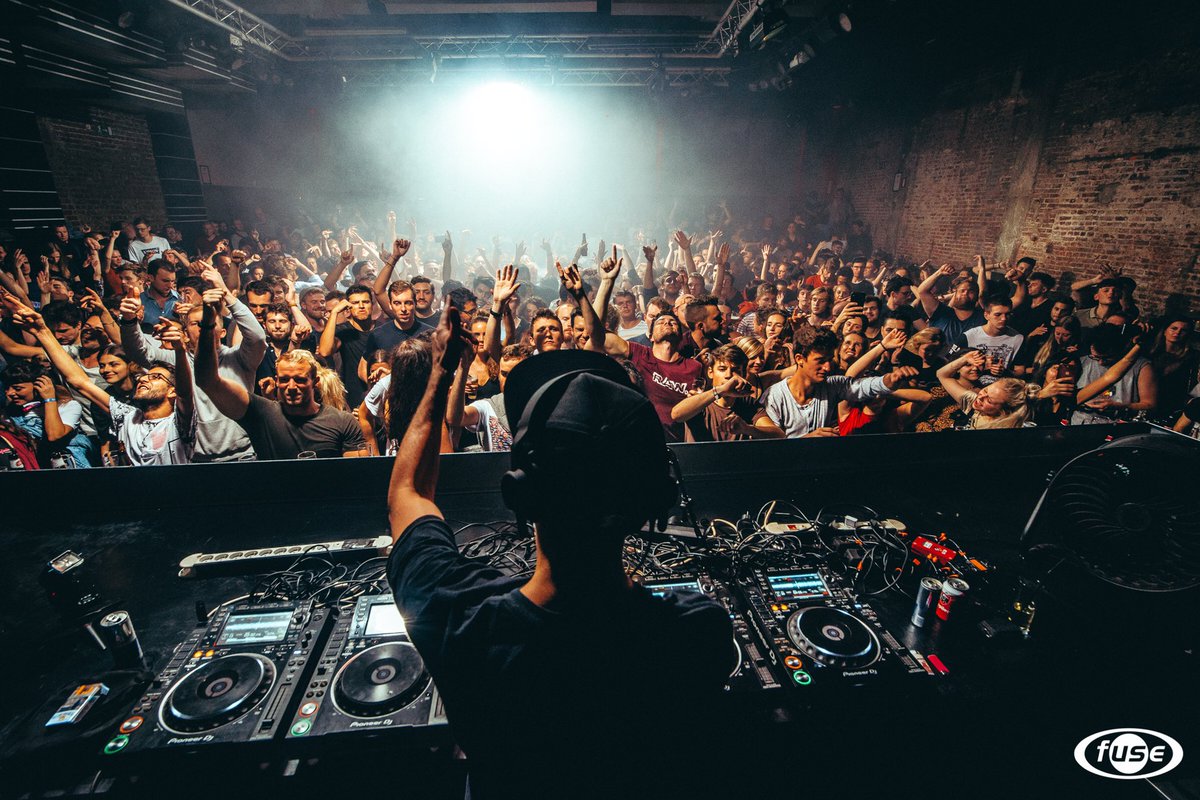The image captures an electrifying scene of a DJ energizing a small, packed indoor venue during a nighttime event. The DJ, donning a headset over his ears, stands behind five turntables entangled with various black wires, hands raised in sync with the enthusiastic crowd. The crowd, with many hands in the air, faces forward, fully immersed in the music. The room, a compact square space with bare red brick walls on the left, right, and back, is filled with around 1 to 200 people. The ceiling, mostly out of the shot, reveals black scaffolding that supports multiple speakers and spotlights illuminating the scene, along with a gray mist emanating from the back ceiling area. The intense white light shining from the background enhances the high-energy atmosphere. In the bottom right corner, a white oval watermark with white letters spells "FUSE," completing the vivid depiction of this captivating music event.